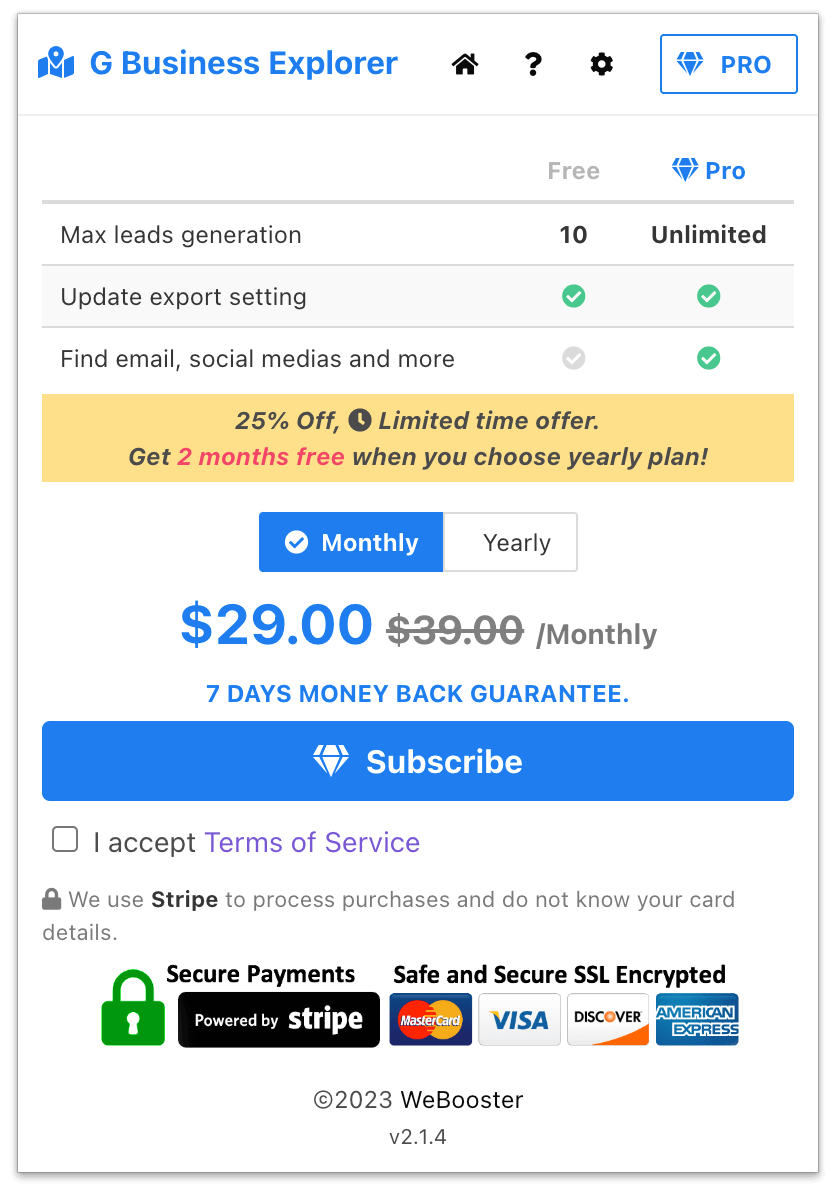This image is a colorful screenshot of a software platform titled "G Business Explorer." The interface prominently features the platform's logo, which resembles an old, unfolded map with a location marker. At the top of the screen are several interactive tabs: "Home", a question mark icon for help and FAQs, and a settings button. 

Below these tabs, the screen displays various subscription options for the product, divided into "Free" and "Pro" plans, with a detailed comparison of their features. The "Free" plan offers a maximum lead generation of 10 and the ability to update and export settings. In contrast, the "Pro" plan provides unlimited lead generation, access to email and social media tools, and additional features.

The pricing for the Pro plan is also showcased: $29 per month with a seven-day money-back guarantee, a reduced price from the former $39 per month. There's an added incentive for users to opt for an annual subscription with a 25% discount, offering two months free. Lastly, a prominent "Subscribe" button accompanies the terms and service agreement link.